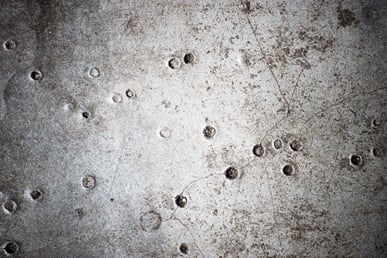This close-up photograph captures an aged, gray metal surface, likely the backdrop of a target practice session or a piece of industrial history possibly displayed in a museum. The entire image is dominated by the metallic texture, showing signs of significant wear, rust, and corrosion, giving it a vintage look. The surface is punctuated by numerous indents and holes, many of which are circular and appear to have been created by bullets. Some bullets seem to have fully penetrated the metal, while others have merely deformed upon impact. These indents are scattered mostly in two rough horizontal lines, suggesting the usage of a submachine gun or similar automatic weapon. Light cracks run through the metal, particularly toward the middle right side, and there's a gradation of color from a silvery light gray at the center to darker hues towards the edges, possibly due to uneven lighting or inherent material variations. The intricate details, including the arrangement and varying depths of the holes, along with the natural and inflicted wear, evoke an image reminiscent of a cratered celestial body or an abstract piece of art imitating such a surface.